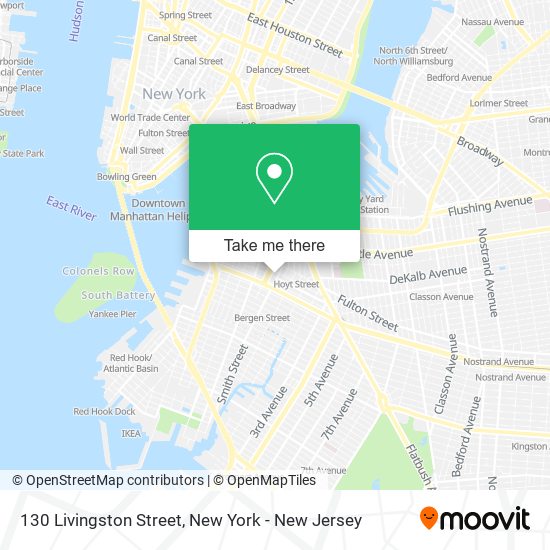In the image, we observe a user interface page from a navigation or transportation software, prominently featuring a detailed map. Located at the bottom right of the page is a distinct logo labeled "MOOVIT," designed as a map pin with a smiling face adjacent to the word spelled M-O-O-V-I-T. Directly to the left of this logo, the address "130 Livingston Street, New York-New Jersey" is displayed, likely indicating the searched destination.

Dominating the upper portion of the page is a detailed map of New York City, complete with labels for significant landmarks such as the World Trade Center, Fulton Street, and Wall Street. Additionally, the map outlines key areas including the rivers surrounding downtown Manhattan and notable locations like the Heliport.

In the middle of the map, a pop-up window showcases an image of a large concrete building, approximately five or six stories high, set against a clear, bright blue sky. This building likely corresponds to the searched address or a major point of interest. The interface seamlessly integrates navigational elements and visual representations to provide a comprehensive users' experience.